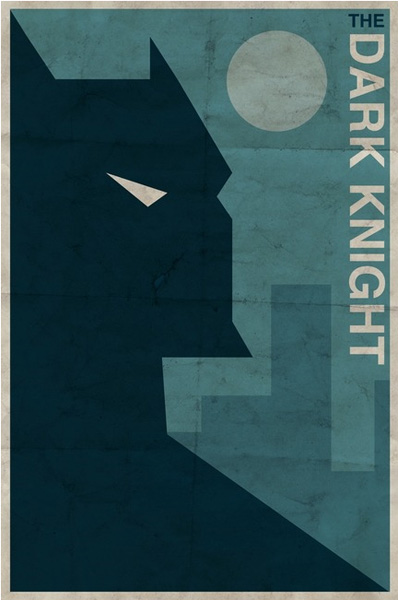The image is a vertically rectangular, minimalist poster featuring a stylized profile silhouette of Batman. A light gray border frames the image, enhancing its clean and simple design. The background is a gradient of blue, transitioning to teal, suggestive of a skyline at dusk, with dark silhouettes of tall buildings peeking out. In the upper right-hand corner of the poster, there's a white moon casting a dim glow over the scene. Text is minimal: the word “The” appears horizontally in black in the upper right, while the words “Dark Knight” are written in white and run vertically along the right side. Batman's profile dominates the left side of the image, characterized by his iconic pointy ears, a sharp chin, and a single eye depicted as a white triangle. The overall aesthetic of the image is dark and shadowy, capturing the mysterious essence of Gotham's vigilante.